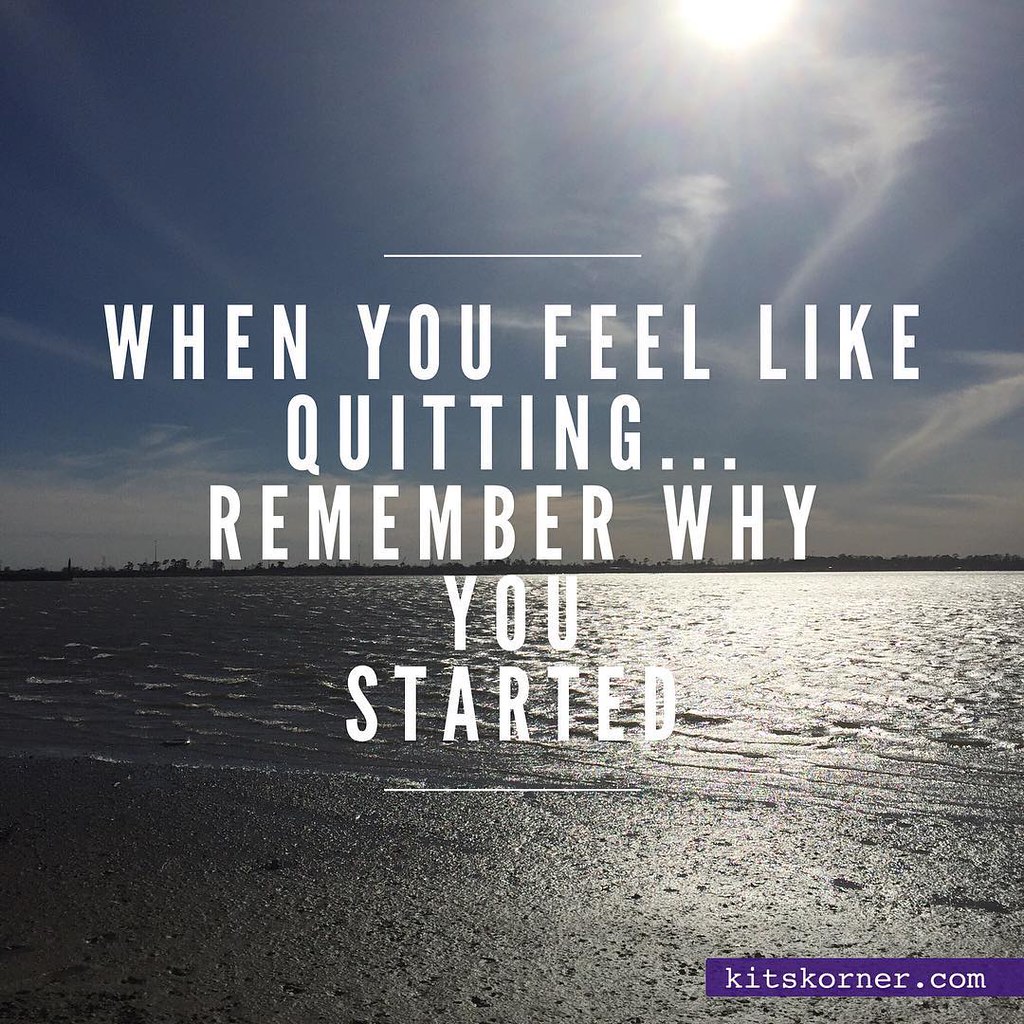The image depicts a serene beach scene with wet sand in the foreground and a relatively calm body of water extending to the horizon. The sun is shining brightly through the wispy clouds in the blue sky, casting gentle light onto the water, which has small ripples. Superimposed across the center of the image in large, white block letters is the motivational quote: "When you feel like quitting, remember why you started." Below this, in the lower right-hand corner, is a small purple banner with the text KitsCorner.com in white.